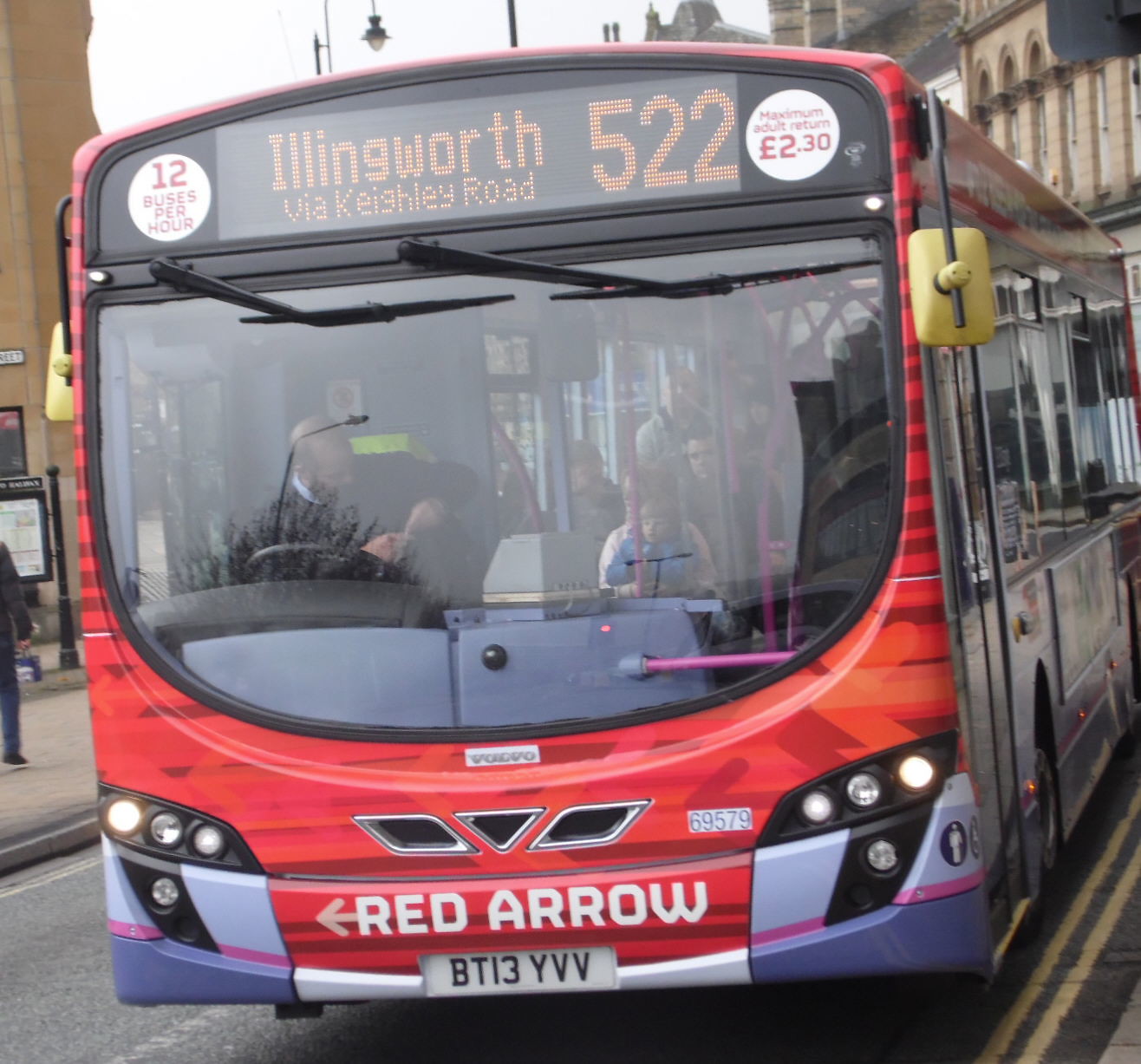This detailed image captures the front of a vividly colored city bus in the UK, specifically marked as traveling to Illingworth via Keighley Road. The prominent red bus features geometric patterns of red, orange, pink, blue, purple, black, white, and gray. At the top, in orange text against a black background, the destination "Illingworth via Keighley Road 522" is displayed, accompanied by a small circular sign indicating "12 buses per hour" and a fare notice, "Minimum adult return 2.30 pounds." The bus is identified by its white-on-red text "Red Arrow" just above the license plate BT13 YVV. The image is a close-up, focusing on the front of the bus, revealing large mirrors on either side, a significant windshield, and detailed views of the bus’s exterior. The male bus driver, with a bald head, is seated on the right and appears to be looking down, indicating the bus might be stationary. The background shows vague snippets of a brick building to the right, a partly cloudy white sky, and part of the curb with a pedestrian visible.